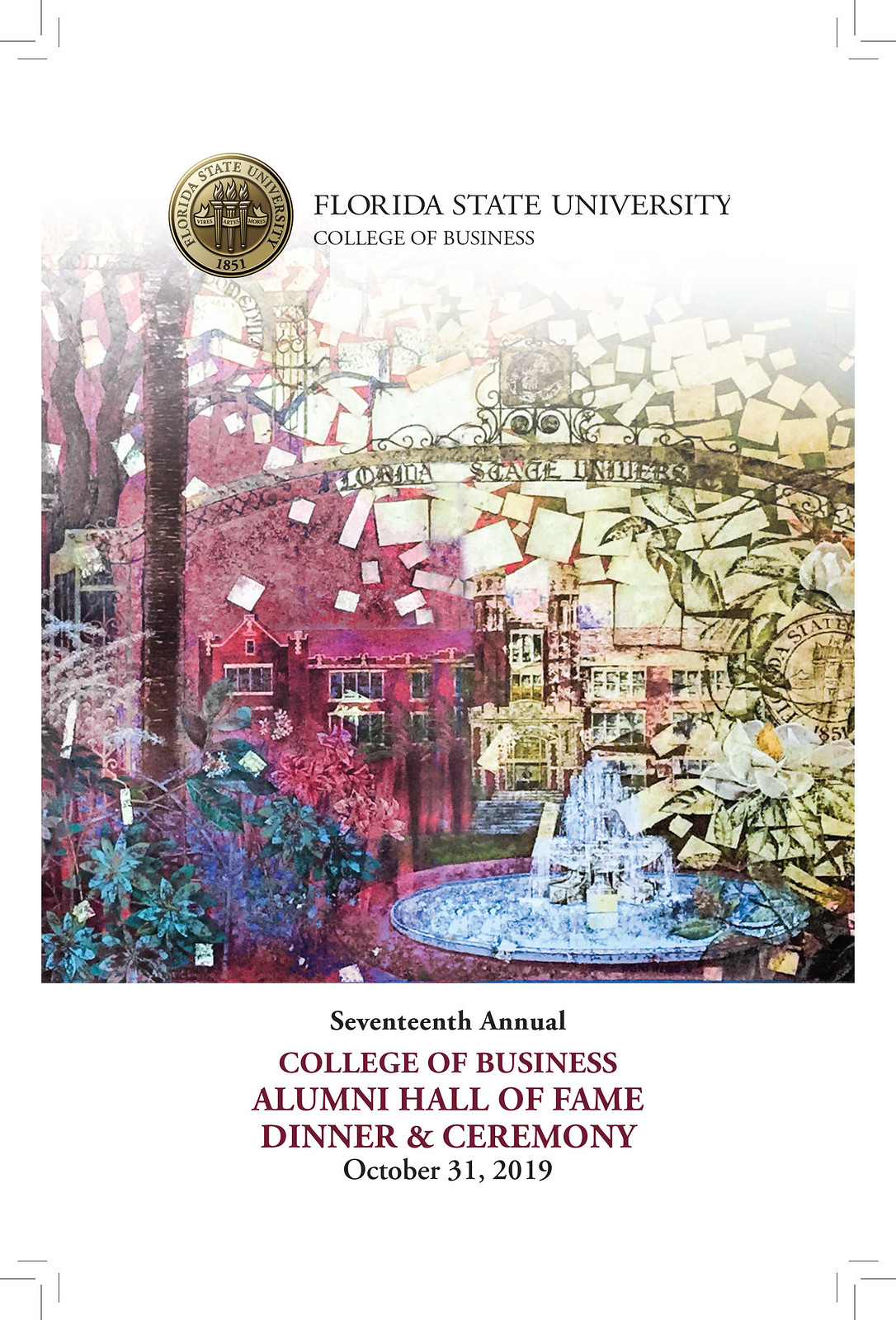The cover image appears to be an artistic, colorful poster or advertisement for the 17th Annual College of Business Alumni Hall of Fame Dinner and Ceremony, held at Florida State University College of Business on October 31, 2019. The top of the image features the text "Florida State University College of Business" along with a round, gold insignia dated 1851 on the left. The central part of the image displays a vibrant, mosaic-like depiction resembling scattered post-it notes, highlighting a blue water fountain amidst an abstract arrangement of squares and floral motifs in yellow, red, blue, and purple colors. In the background, there is a series of buildings, including a prominent yellow one and a pink wall with windows cut out, alongside some foliage and a tall tree trunk. Below the mosaic, additional text in black and brown announces the event details: "17th Annual College of Business Alumni Hall of Fame Dinner and Ceremony."